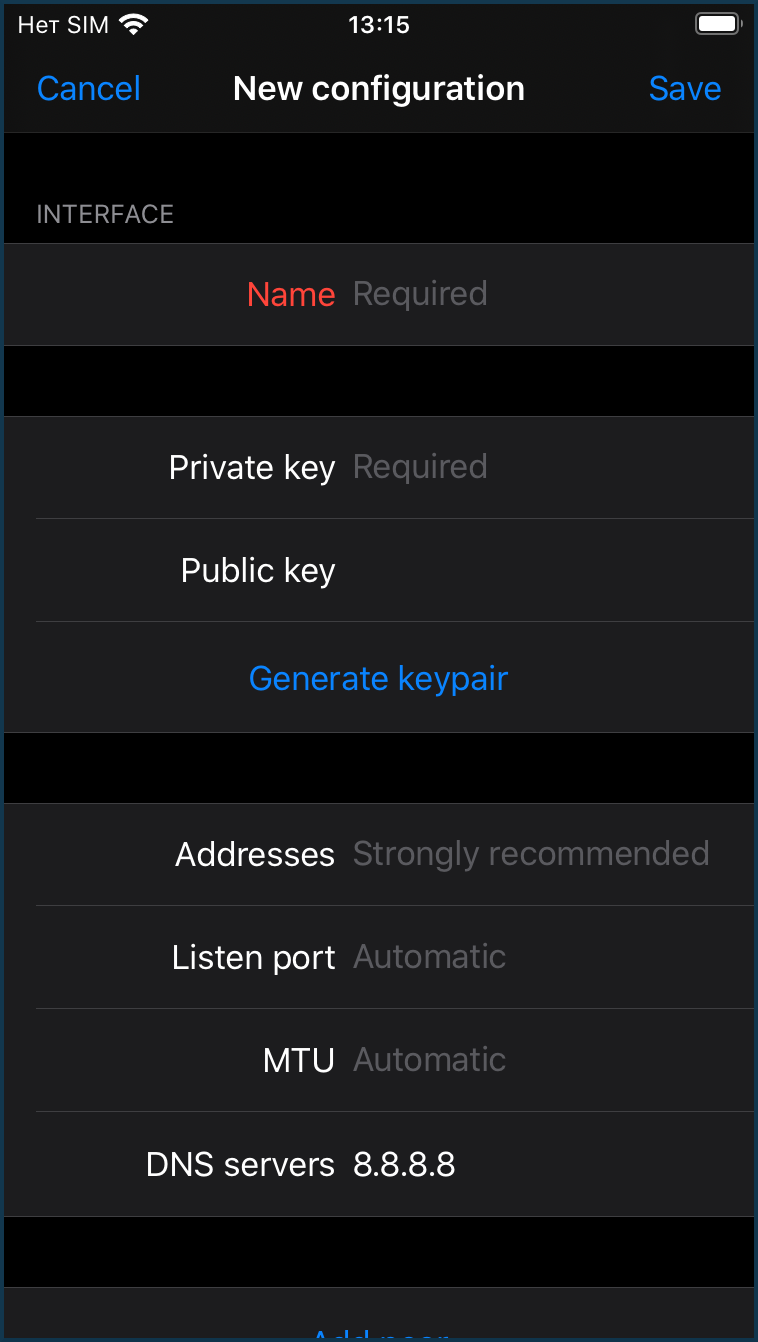The image displays a mobile phone screen with a black background, indicating it’s from a screenshot. Starting from the top left corner, there is the text "HET SIM" alongside a Wi-Fi or cell signal icon. Centered at the top is the time, marked as 13:15, and in the upper right corner, there's a fully charged battery icon.

Below this status bar, the screen shows options presumably part of a new network configuration setup. At the top of the setup section are three buttons: "Cancel," "New Configuration," and "Save," with "Cancel" and "Save" being highlighted in blue, suggesting they are actionable options.

The fields to be filled out in the configuration form include:

1. **Interface**:
   - "Name Required" (text in red)
2. **Keys**:
   - "Private Key Required"
   - "Public Key" with an option to "Generate Key Pair" (the actionable button in blue)
3. **Network Settings**:
   - "Address" (marked as "strongly recommended")
   - "Listen Port" (default setting is "Automatic")
   - "MTU" (default setting is "Automatic")
   - "DNS Servers" with the IP "8.8.8.8"

All headings (like "New Configuration," "Private Key," "Public Key," "Address," "Listen Port," "MTU," and "DNS Servers 8.8.8.8") are in white. Additional descriptive texts (such as "required," "strongly recommended," or "automatic") are displayed in grey, making the main and supplementary information clearly distinguishable.

The layout is designed for clarity and ease of understanding, guiding the user to either complete the form and save the configuration or cancel the operation if they choose.